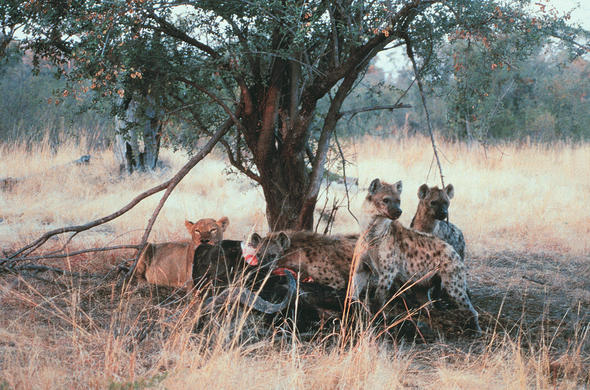In this soft-focus, dusk-colored photograph, we see a dramatic scene unfolding in a dry, sunlit environment that resembles both a jungle and a grassland. The center of the image is dominated by a small wiry tree with sprawling branches and small green leaves, casting shadows over the animals beneath it. Upon closer inspection, we notice a lioness reclining in the shade next to a fallen branch. Nearby, three spotted hyenas stand, with two appearing alert and looking off into the distance while the third is engrossed in eating what seems to be a dead yak. The golden, bronze hues of the sunset or dusk light accentuate the dry grass and soil, emphasizing the harsh yet captivating atmosphere of the landscape. Overall, the image blends elements of photorealism with a softer, painterly aesthetic, heightening the dramatic interaction among the predators.